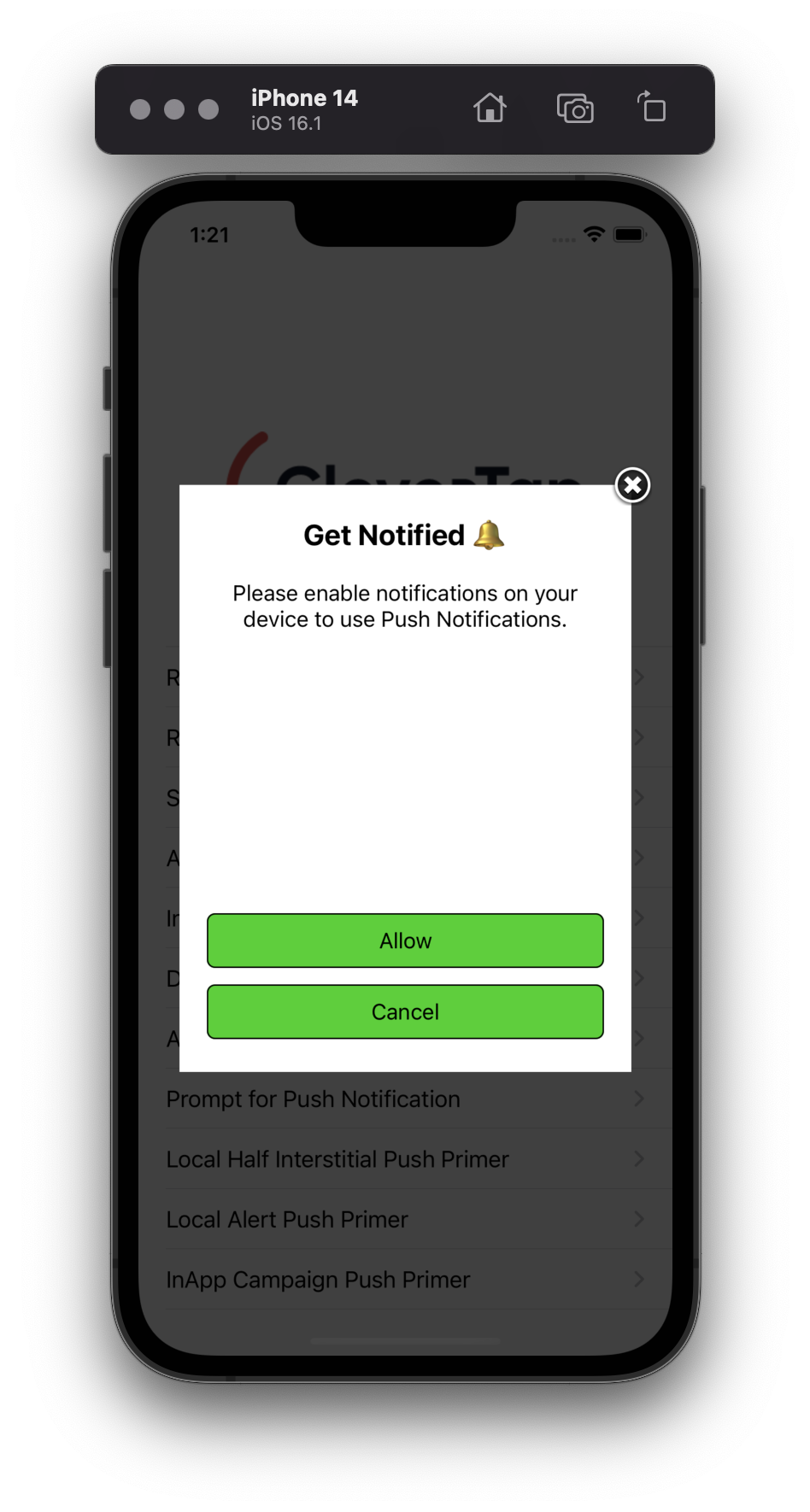The image displays a graphic representation of an iPhone 14 running iOS 16.1. The main focus is on the phone screen, which shows a dark background with a prominent white pop-up notification box. This notification prompts the user to "Get notified. Please enable notifications on your device to use push notifications." Below this message, there are two buttons: a green "Allow" button and a green "Cancel" button. Overlaid at the top of the phone image is a separate dark-colored box featuring three icons: a home icon, a photos icon, and a square-shaped icon on the far right. Despite the pop-up covering the majority of the screen, some underlying options are partially visible, including "Prompt for push notification," "Local half interstitial push primer," "Local alert push primer," and "In-app campaign push primer."